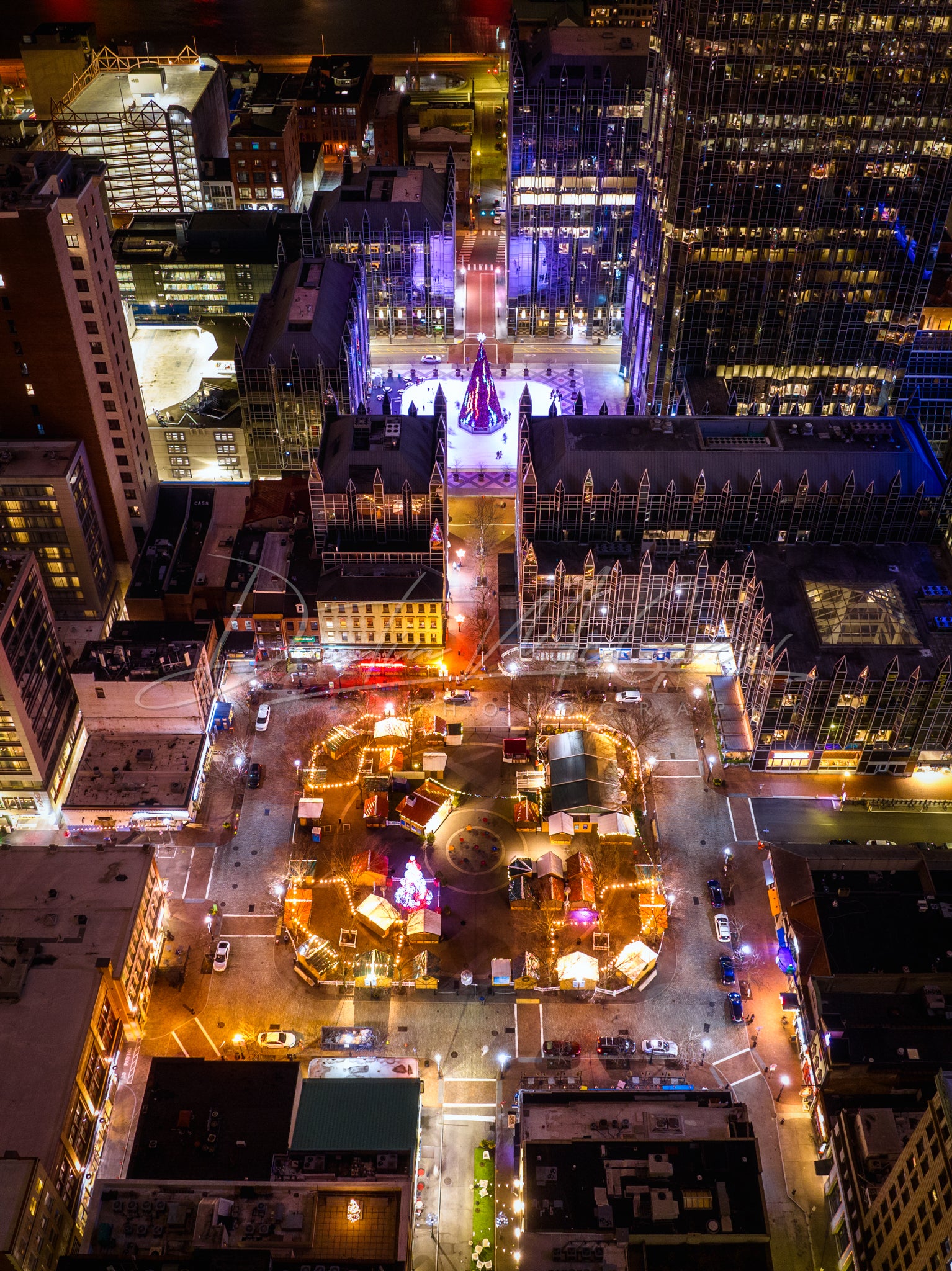An aerial view of downtown Pittsburgh at night highlights a vibrant and picturesque cityscape. The brilliantly lit skyline is adorned with high-rises of varying heights, their windows aglow with office lights. A central focal point of the image is Market Square, a circular plaza bustling with activity. The square hosts ornately decorated buildings and vehicles parked neatly in front of them. Illuminated streets crisscross through the area, their lights creating a network of glowing pathways.

In the middle of the square, there appears to be an ice-skating rink, encircled by shed-like structures resembling Christmas stalls. These are beautifully adorned with twinkling lights, contributing to the festive ambiance. A splendid conical Christmas tree, decorated and brightly lit, stands out in the distance in another secondary square, adding to the holiday spirit.

Further aspects of the downtown area include various cubic rooftops viewed from above, parking lots with neatly arranged cars, and a vividly lit parking garage. The overall scene provides a captivating and detailed view of a city alive at night, with its architectural grandeur and holiday decorations creating a truly beautiful image.